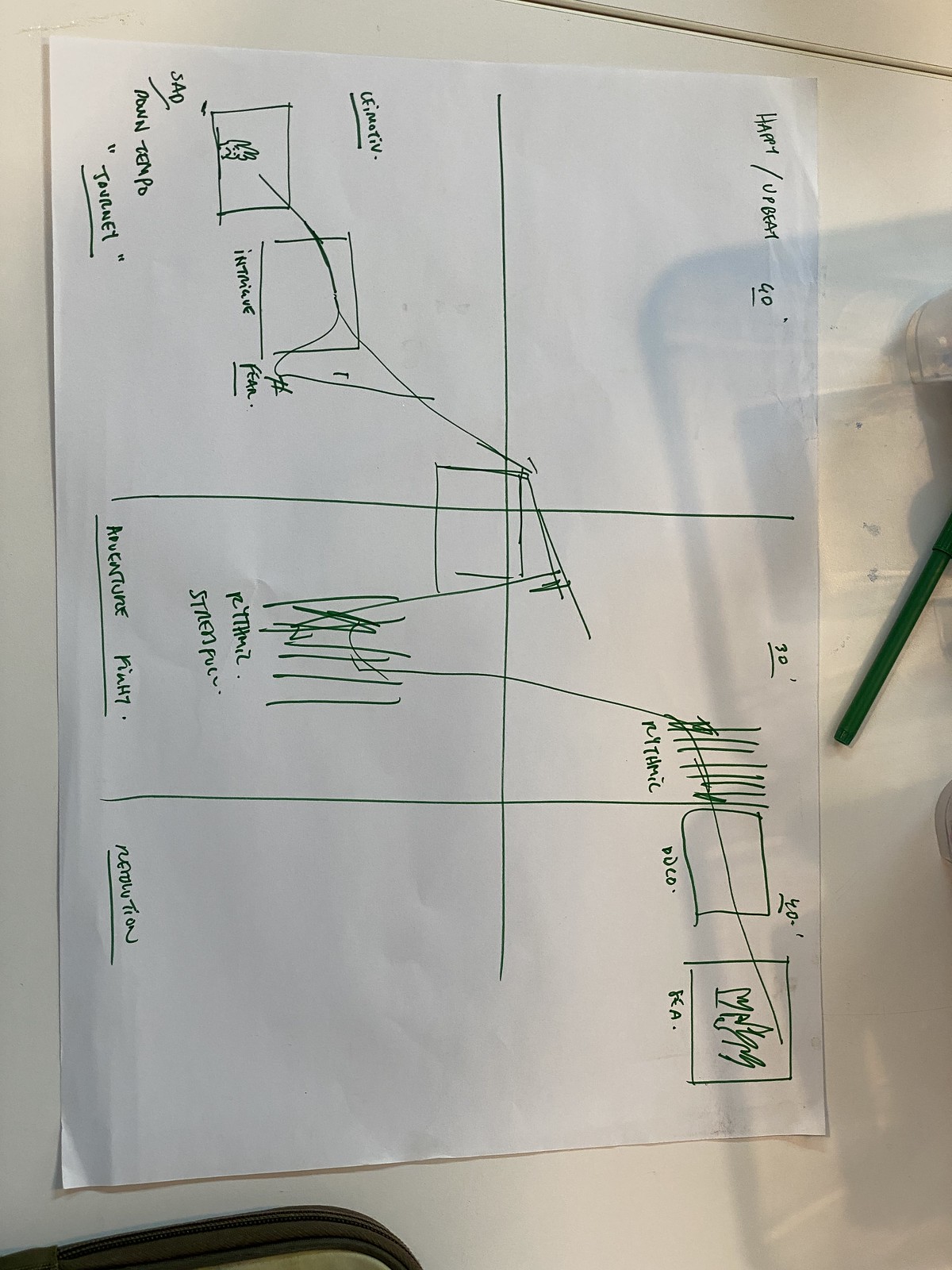The photograph features a white piece of paper, either photographed from above laying flat on a white table or mounted on a wall; the angle and surroundings make it ambiguous. The paper is divided into six equal rectangles by one central vertical line and two horizontal lines. The left column of the paper contains writing and underlines in each of its three sections, although the text is illegible and resembles scribbles.

In more detail:
- The top left square has small squares with lines intersecting them and some random doodles in the center.
- The middle left square is filled with more scribbled lines.
- The bottom left square is mostly blank with minimal markings.

The right column of the paper appears more organized:
- The top right square has tally marks, as if counting something.
- Both the middle and bottom right squares also feature similar tally marks.

Additionally, a prominent black diagonal line crosses the right middle section of the paper, extending from near the center bottom to the middle right edge.